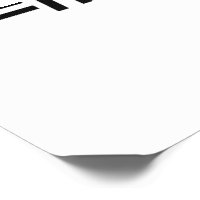The image depicts a slightly lifted white piece of paper positioned diagonally towards the viewer on a white surface, causing shadows under the upturned corner. The lighting is flat, merging the paper with the background. In the top left corner of the paper, there are distinct black lines: a thin diagonal line moving from top right to bottom left, a thicker horizontal line moving rightward from the left, a vertical bar crossing down near the edge, and another bar peeking in from the right. The bottom of the page features a complex thin line emerging from the left, angling down and broadening into a wide, flat, circular shape in the center before narrowing and extending off the page to the right. The lines and shapes suggest some form of abstract or minimalistic design.